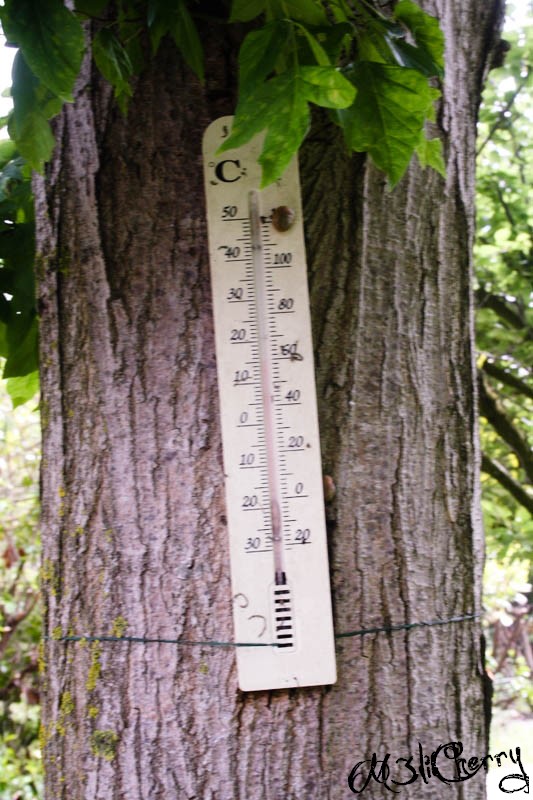A thermometer is securely strapped to the trunk of a tree, measuring the ambient temperature. The thermometer features a wooden casing, which serves as a rustic backdrop for the instrument. On the bottom right corner of this casing, there's an artist's signature reading "M3LI Cherry." 

The thermometer displays two scales: the left side is marked in Celsius with intervals from -30 to 50 degrees, and the right side is marked in Fahrenheit with intervals from -20 to 120 degrees. Currently, the temperature reads approximately 60 degrees Fahrenheit (15 degrees Celsius). Surrounding the thermometer are vibrant tree leaves, suggesting a lush, outdoor environment. The image is taken during daylight, highlighting the natural setting and providing a clear view of the thermometer’s details.